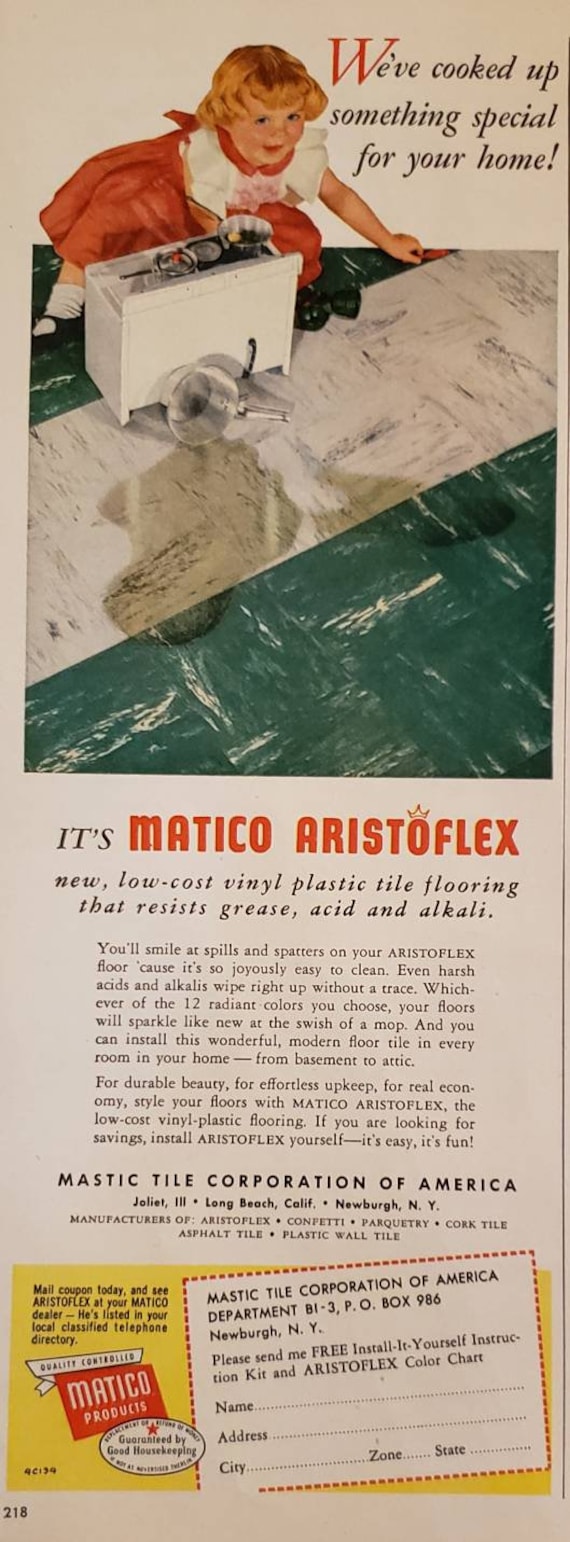This vintage magazine advertisement for Mestico Aristoflex showcases a young girl with curly reddish-blonde hair, dressed in a red and white dress, red collar, white socks, and black Mary Jane shoes. She is kneeling on a teal and white marble-patterned tile floor, from which a boiling pot of water has fallen, spilling liquid across the tiles. The text at the top reads, "We've cooked up something special for your home," highlighting the durability and aesthetic appeal of the new low-cost vinyl plastic tile flooring, which resists grease, acid, and alkali. Beneath the image, it features the text "Mestico Aristoflex" and mentions the Majestic Tile Corporation of America. The bottom of the ad includes a cut-out coupon for requesting more information.